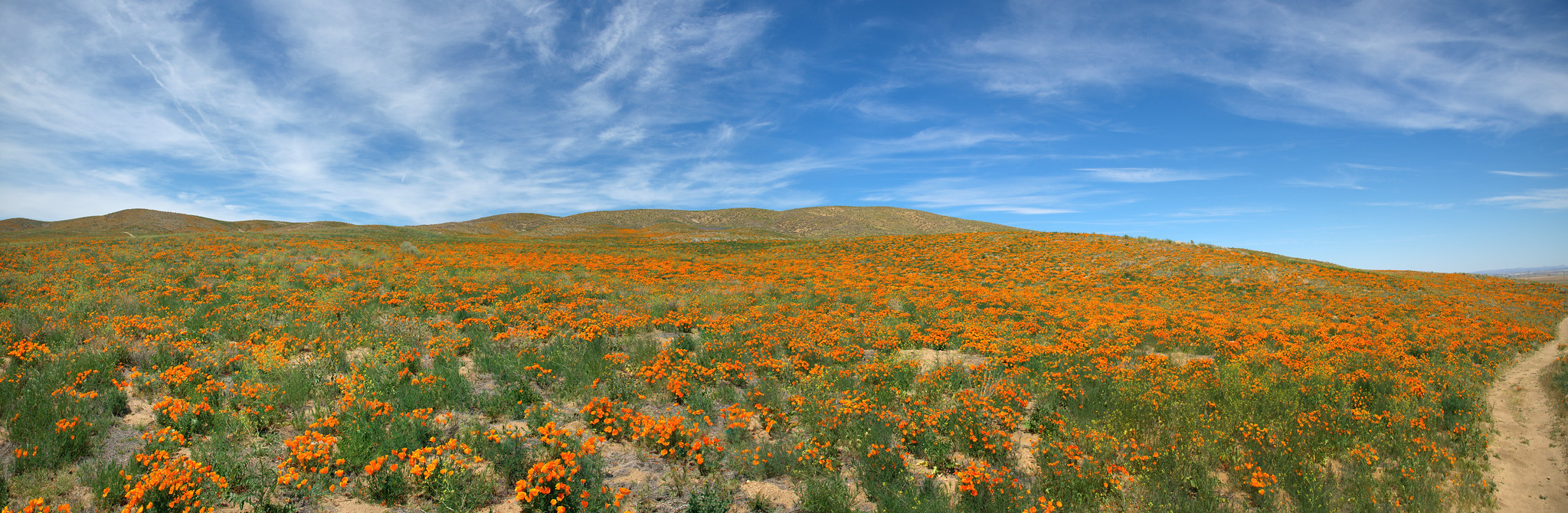This vibrant, wide-aspect color photograph captures a picturesque landscape with captivating detail. In the foreground, a sea of vibrant orange flowers blooms amidst patches of earthy grass, interspersed with areas of tall, lush green grass. As your eye moves towards the background, the landscape gently transitions into rolling hills, creating a sense of depth and tranquility. The sky overhead is a crisp, serene blue, adorned with numerous thin, wispy clouds that stretch across the horizon. On the far right, a meandering trail starts from the bottom right corner and curves delicately to the edge of the image, inviting one to ponder the journey it promises. The scene is devoid of any human or animal presence, buildings, vehicles, or any modern intrusions, allowing nature's raw beauty to take center stage.